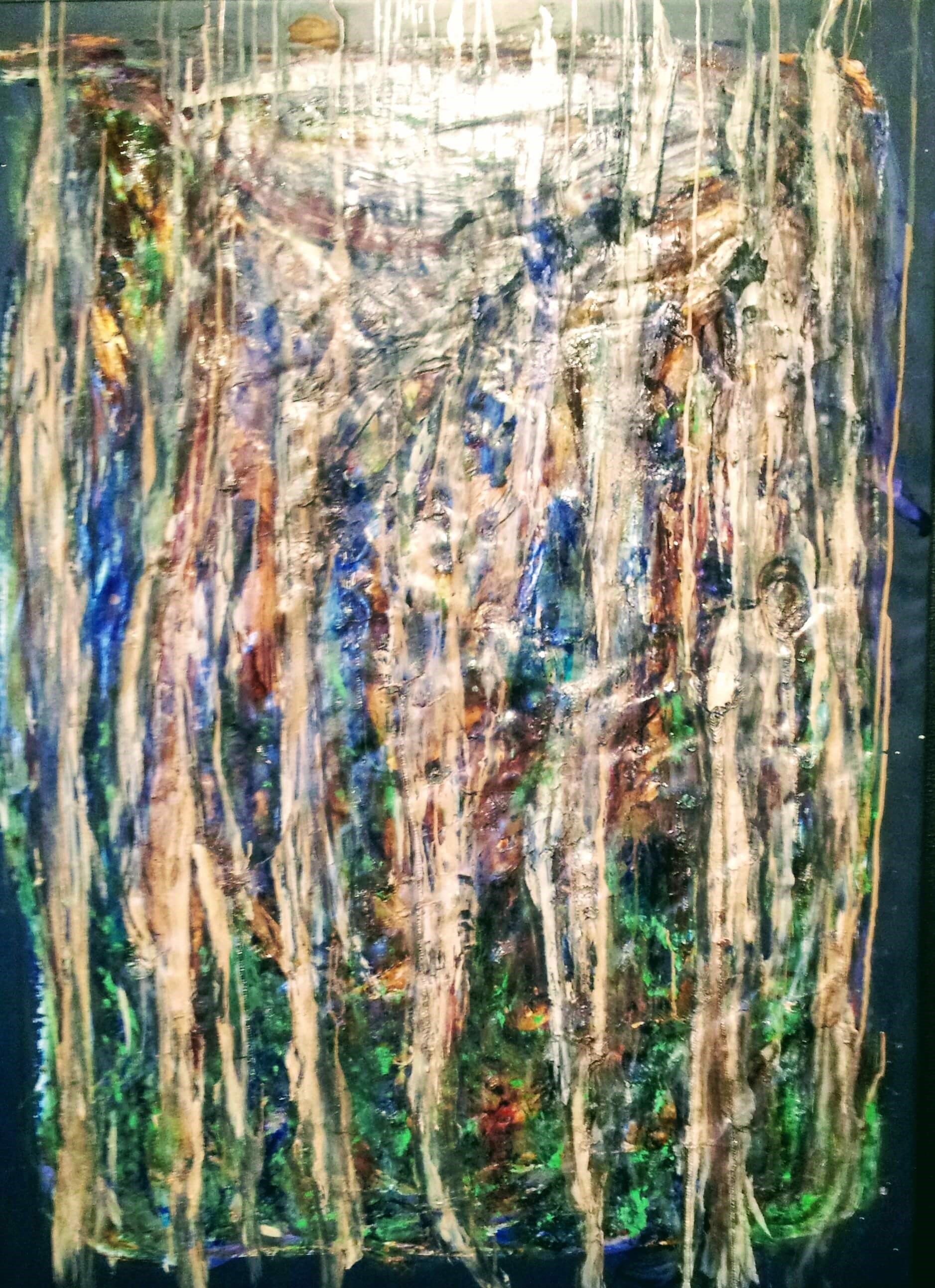This painting features a mesmerizing array of vertical streaks that resemble elongated roots cascading from top to bottom, set against a black background. The strokes incorporate a palette of diverse colors including shades of green, blue, gray, white, brown, and metallic gold. The streaks are irregular and seem to convey more than just abstract forms; vague impressions of eyes and partial faces are subtly embedded within the lines, invoking a sense of hidden, enigmatic figures. At the bottom, the streaks transition into a grass green hue while they fade into a lighter, milky white at the top. The overall effect is enhanced by the appearance of the streaks shimmering as if viewed through a layer of saran wrap, adding a further layer of intricacy and texture to the compelling visual narrative of the piece.